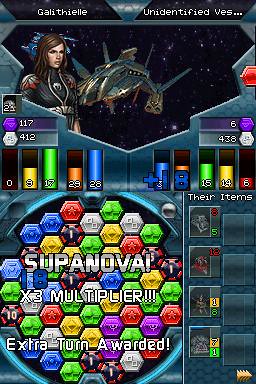This image depicts a screenshot from a low-quality mobile match-3 video game called "Galithiel." Dominating the screen's upper section, the title "Galithiel," followed by the phrase "unidentified vessel" is displayed in white lettering alongside a metallic triangle symbol. 

To the left, various stats are shown: a purple stat of 117 and a white stat of 412. On the right side, stats include a purple 6 and a white 438. Below the title, there is a graphic of a Star Trek-style female character with long dark hair positioned in front of a window viewing outer space and a spaceship.

Centrally, the gameplay area is designed with hexagonal shapes resembling a beehive, colored in red, green, purple, yellow, white, and silver, along with some mixed colors like black and red. Above this area, in bold text, it says "Supernova times three multiplier, extra turn awarded."

Flanking this central space are various color-coded bars filled with different liquid levels. On the left, bars contain blue, orange mixed with blue, green, yellow, and red liquids. The right side mirrors these colors, reinforcing the competitive nature of the game. This blend of colorful hexagons and liquid-filled bars outlines the game's primary mechanics, evidently a match-3 puzzle format.